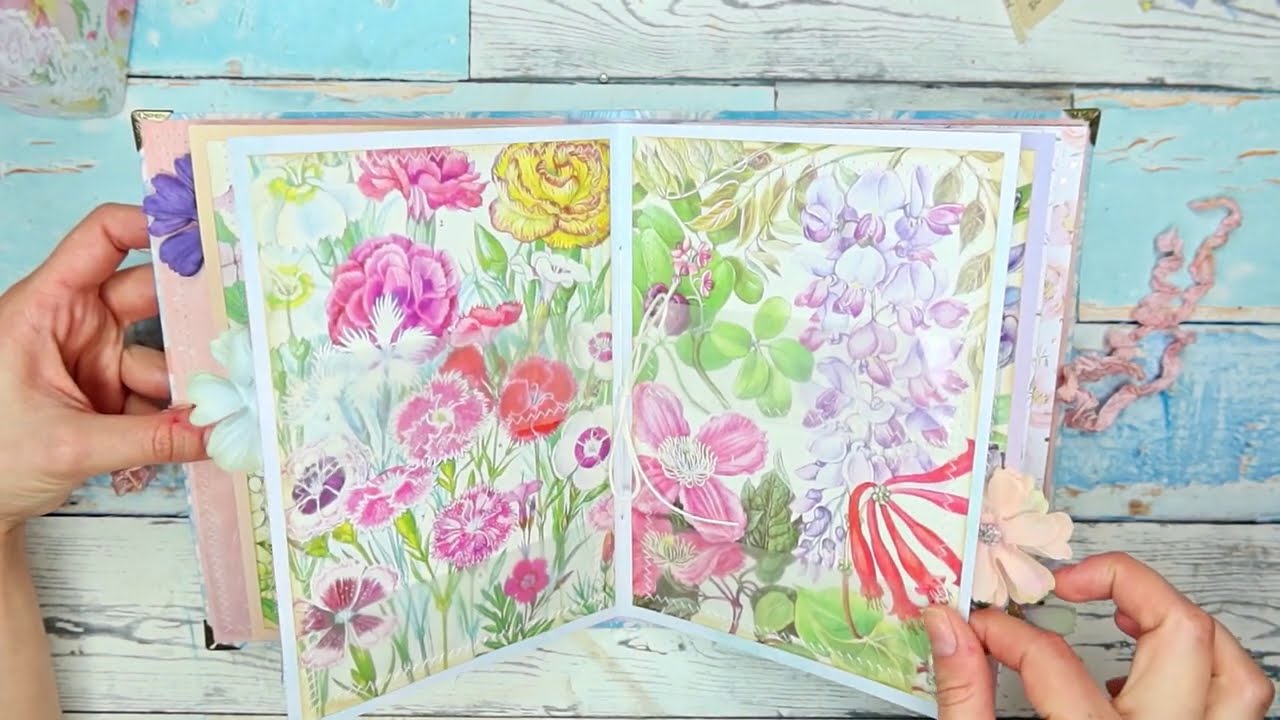The image is an overhead view of a detailed scrapbooking or journaling example, set against a weathered, pale blue and gray wooden background that evokes a coastal, weather-beaten vibe. In the center of the image, a pair of woman's hands are holding open a book, showcasing its vibrant, watercolor-painted pages. Each page is adorned with an array of colorful floral illustrations including yellows, pinks, reds, purples, and greens, representing various plant species. The book also features 3D flower accessories interspersed amongst the pages, adding depth and texture to the artwork. The intricate design and diverse colors of the flowers make the book not just a journal but an art piece in itself, filled with delicate, rainbow-hued botanical illustrations and real flower elements carefully tucked between the pages.